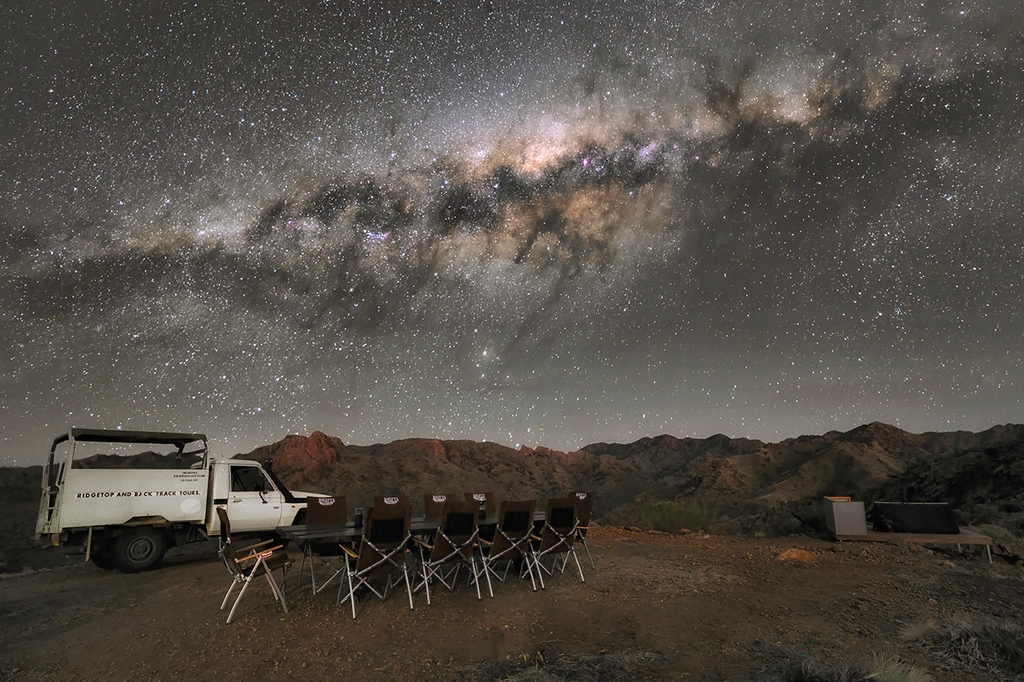In the image, a white truck with the words "Bridgetop and Back Truck Tours" is parked on the left side of a rocky, red desert landscape. The bottom third of the image features this rugged terrain, along with a long black table set up in front of the truck. Surrounding the table are ten brown folding camping chairs, with eight positioned along the sides and one at each head, creating a setup that seems ready for an outdoor gathering. To the far right of the image, a small black tent and a gray wind blocker device are noticeable. The top two-thirds of the image are dominated by a mesmerizing and vibrant view of the Milky Way Galaxy. The night sky is densely scattered with stars, showcasing colors such as black, yellow, orange, and brown. This breathtaking galaxy image spreads across the entire sky, adding a celestial depth and allure that captivates the viewer's eye.